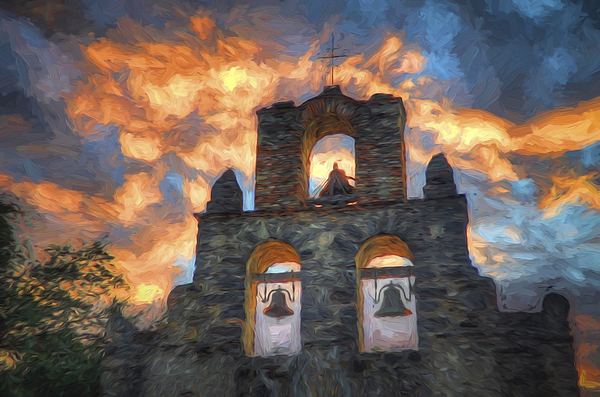The image showcases an oil-on-canvas painting depicting the top of an old stone mission building, likely a church. The structure features two lower arched windows, each housing dark gray bells suspended by a bar near the top. Above these, there's a third arched window with an additional bell and the subtle silhouette of a person in a white dress. Standing above this section is a thin cross. The sky behind the building is a striking blend of vivid colors: fiery yellow, medium orange, and dark orange hues suggest a dramatic evening sky, interspersed with dark and light blue sections along with some gray and white clouds. The lower left corner of the painting is adorned with dark green shrubbery, adding a touch of nature to the scene. The overall atmosphere suggests an ancient, serene ambiance backlit by the brilliant, almost chaotic display of the setting sun.